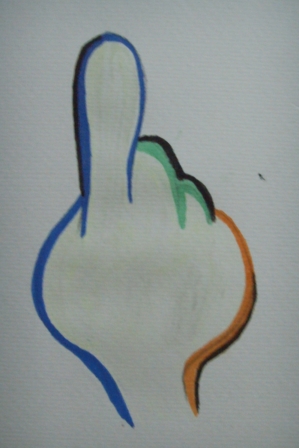This photograph captures a drawing on a white surface, featuring a stylized, playful depiction of a hand with its index finger pointed upwards, symbolizing a gesture of attitude. The hand is illustrated with different colors: the thumb and the left side of the hand, including the pointer finger, are drawn with a blue line that transitions into a green outline for the middle and ring fingers. The final, little finger and the right side of the hand are detailed with an orange line, all bordered with a black outline. The hand is clenched into a fist except for the extended index finger. The image overall gives off a youthful, non-realistic vibe, with dimensions similar to a magazine page.